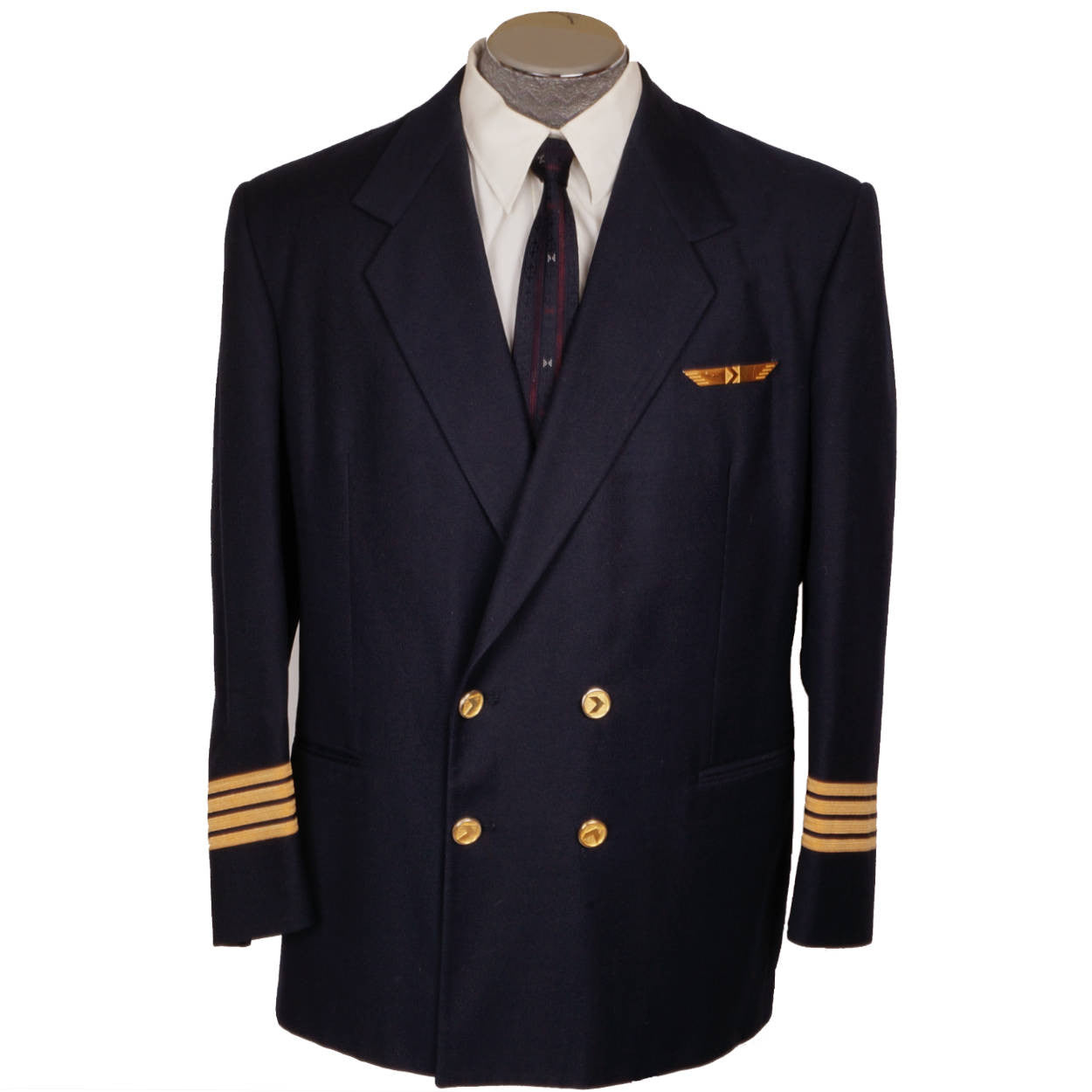This professionally staged full-color photograph features a vertically rectangular image of a vintage-style pilot's uniform. The background is completely white, offering a clear contrast to the navy blue jacket displayed on a headless mannequin, with its neck peeking out of the white dress shirt. The jacket is adorned with four circular gold buttons, each featuring a right-facing arrow, and bears four gold stripes on each sleeve, denoting rank. A set of pilot’s wings pin is affixed to the left breast pocket, complete with a right-facing arrow in the center. The ensemble is completed with a dark blue and red striped tie displaying two small white H's and a crisp white collared shirt underneath. The photograph captures only the torso of the mannequin, focusing solely on the jacket, shirt, and tie, making it a standout representation of the pilot's uniform against the stark white backdrop.